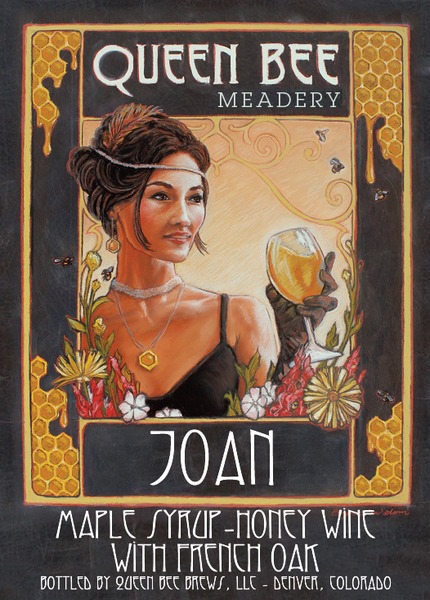The poster for Queen Bee Meadery prominently features an illustration of a sophisticated woman named Joanne. She is depicted with short dark hair, styled with a feather, and is adorned with intricate accessories, including a choker and a long necklace with honeycomb-designed pendants. Joanne is elegantly dressed in black, wearing gloves, and holding a glass of yellow-colored mead. Her face is beautifully made up, and bees hover around her forehead, complementing the honeycomb motifs present throughout the image. The background is filled with depictions of bees, flowers, and honeycombs, enhancing the thematic elements. The top of the poster displays the name "Queen Bee Meadery," and below Joanne, it reads "Maple Syrup Honey Wine with French Oak," followed by the note "bottled by Queen Bee Brews LLC, Denver, Colorado."